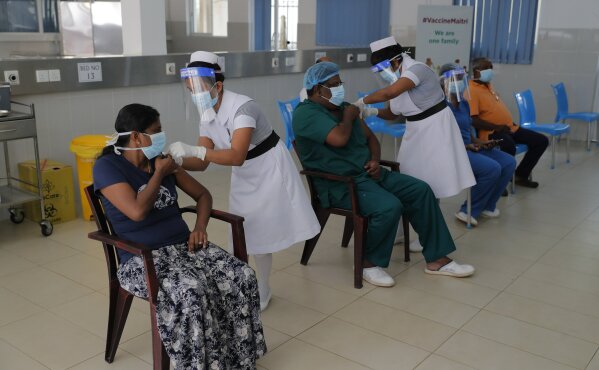The photograph captures a medical setting, likely within a hospital or clinic, where multiple people are receiving COVID-19 vaccinations simultaneously. The scene is rectangular, with the long sides twice the length of the short sides. There are rows of blue chairs, each occupied by an individual receiving a vaccine from nurses. The nurses are dressed in traditional white and gray uniforms, complete with plastic face shields, blue and white face masks, latex gloves, white tights, and white shoes. Each recipient has their left arm exposed, ready for the injection. The floor is covered with large, rectangular white tiles, and a low wall with a metal railing is visible in the background. Blue curtains hang over the windows. 

Across the back of the room, a large sign reads "#VaccineMatri We are one family," indicating a communal effort. The overall environment underscores the systematic and organized approach to the vaccination process. All individuals, both nurses and recipients, appear to be of Indian descent, reinforcing a sense of community and solidarity in this public health initiative.